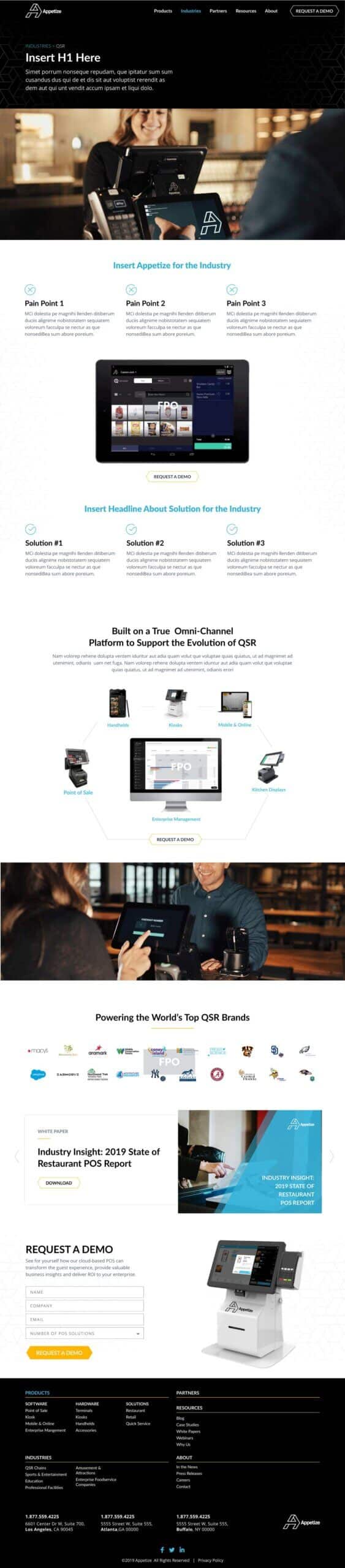This image depicts a promotional flyer for a cash register machine. The document is filled with numerous small paragraphs of detailed information, making it challenging to read. The layout includes several sections, each containing text that appears to describe the features and functionalities of the machine. Additionally, there's a designated area where interested parties can fill out their information to request a demo. Alongside the text, the flyer features a couple of images showcasing the cash register machine in action. The overall design suggests a professional marketing effort aimed at conveying the benefits and usability of this particular cash register model.